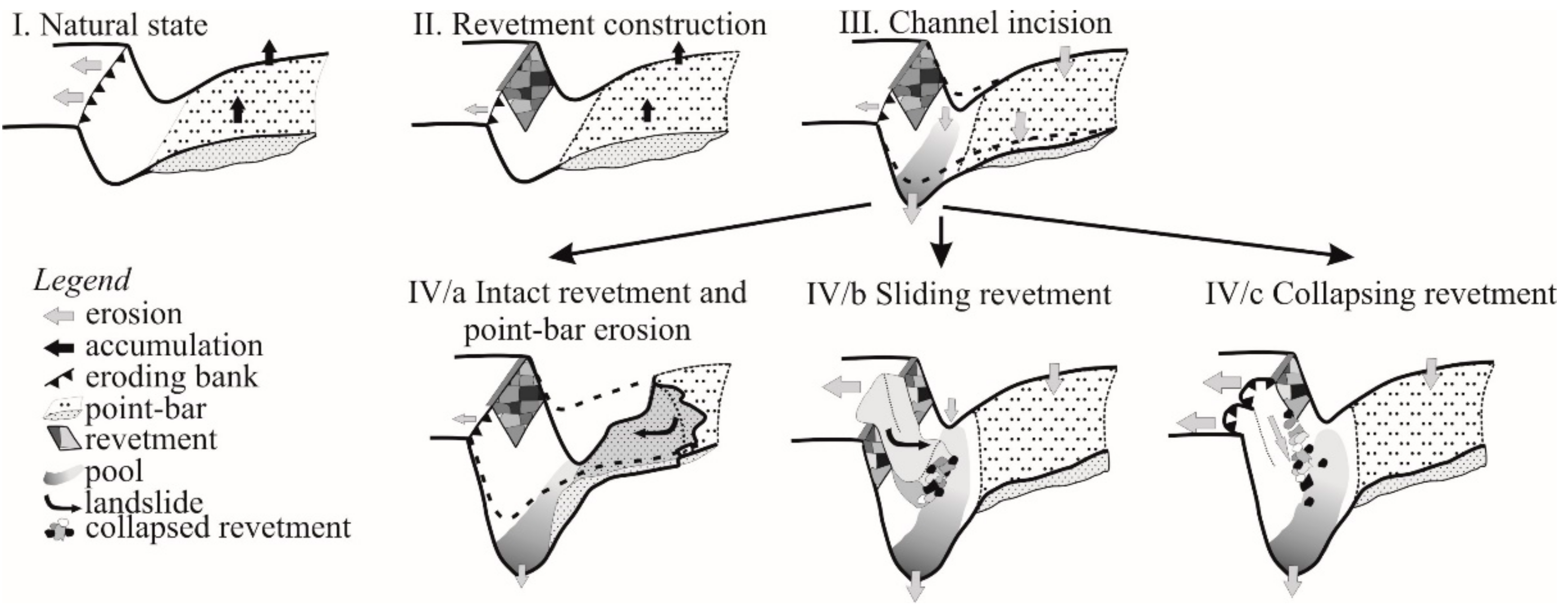The image is a detailed diagram against a white background, featuring four primary sections labeled with Roman numerals and a comprehensive legend in the lower left corner. In the upper left is "I. Natural State," accompanied by a black and white image depicting the land in its untouched condition. Moving to the upper middle, "II. Revetment Construction" is shown with a corresponding image. The upper right corner features "III. Channel Incision," along with another black and white image. Below these, in the central lower part, there's "IV.A. Intact Revetment and Point Bar Erosion," leading to "IV.B. Sliding Revetment" immediately to its right, and "IV.C. Collapsing Revetment" further to the right. Each image is marked with arrows and dotted lines indicating various geological or erosional processes. The legend in the lower left corner defines the symbols used: a light gray arrow for erosion, a dark black arrow for accumulation, along with keys for eroding banks, point bars, revetments, pools, landslides, and collapsing revetments. The diagram illustrates different stages of land development or geological change, likely related to erosion and construction processes seen in geology textbooks.